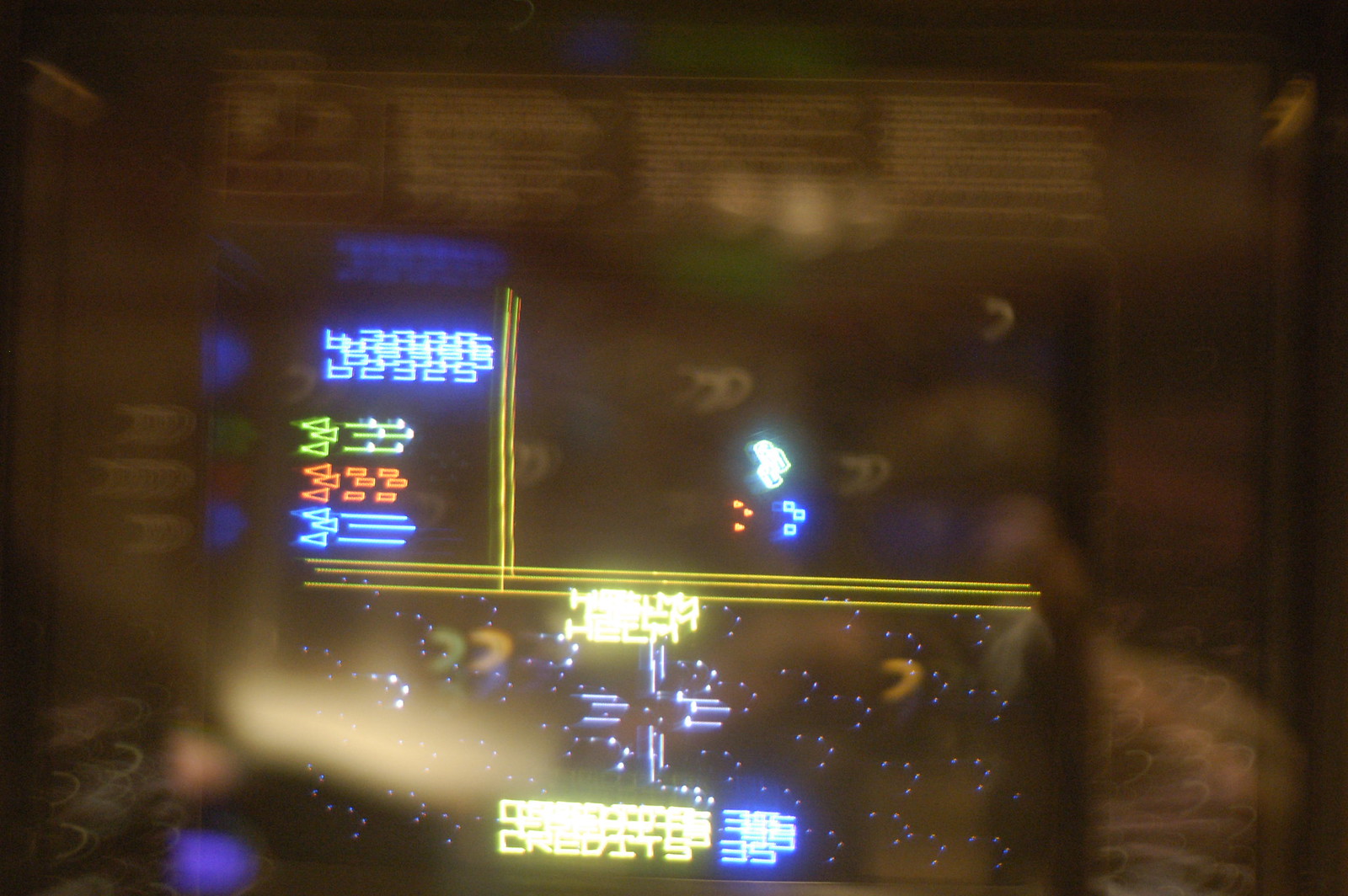A heavily blurred photograph captures the central screen of an arcade game, framed by the decorative border of the arcade cabinet. The screen is brightly illuminated with vibrant colors, including blue, green, red, and yellow. The image is divided horizontally with a yellow line, and a vertical yellow line intersects the horizontal one about a third of the way across. In the upper left corner of the screen, a set of indistinct numbers is displayed. Scattered around the screen are green, red, and blue triangles and lines, along with red, green, and blue dots forming patterns. Below this, a section features stars and a credit display indicating the number 35.